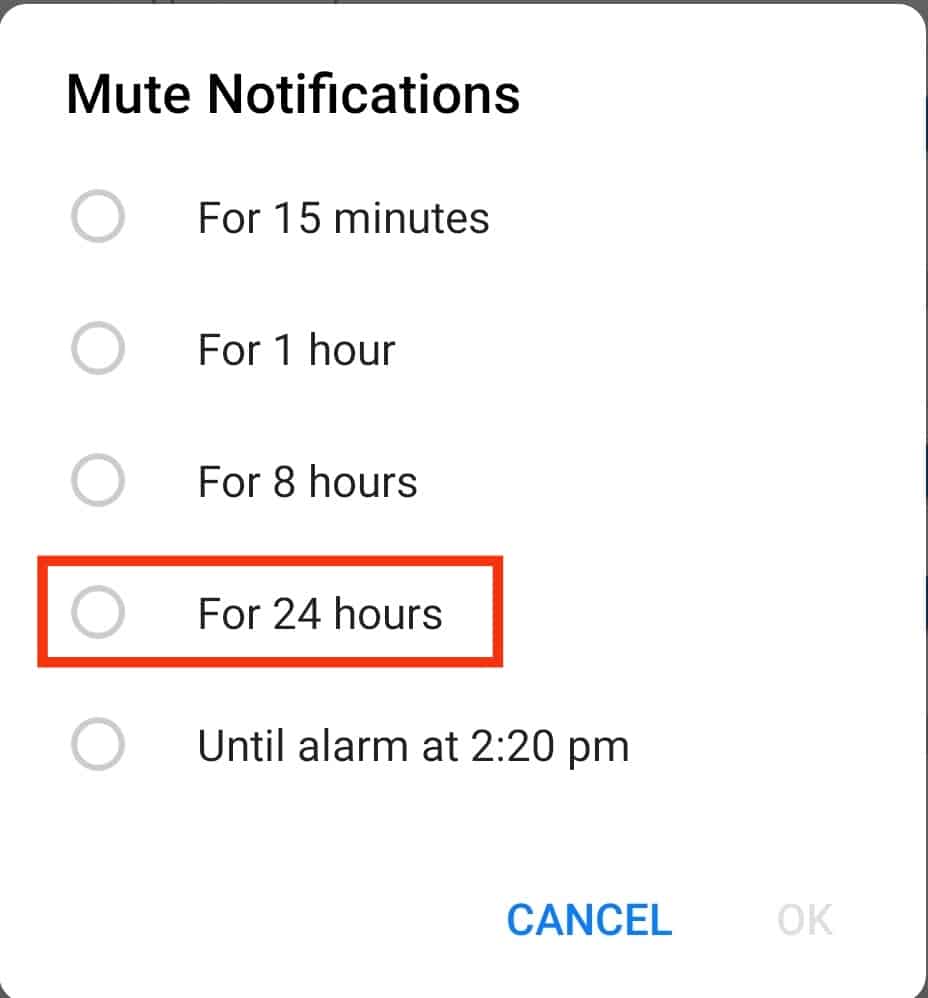This image is a cropped screenshot of the notifications mute options from a mobile device. The screenshot focuses solely on the section labeled "Mute notifications." On the left side, a series of bubble-like radio buttons offer different duration choices for silencing notifications. The options available are:

- 15 minutes
- 1 hour
- 8 hours
- 24 hours
- Until alarm at 2:20 PM

At the bottom of the screen, options to "Cancel" (in blue font) and "OK" (in gray font) are displayed, indicating that an option needs to be selected before proceeding with "OK." Notably, the "24 hours" option is highlighted with a red rectangle, suggesting it is either the preferred or example selection. Despite this highlight, all the radio buttons remain in their default gray state, indicating none have been actively selected yet.

The corners of the screenshot are slightly cut off, bordered by a gray frame, implying that the image has been cropped from a larger screenshot of the phone's screen.